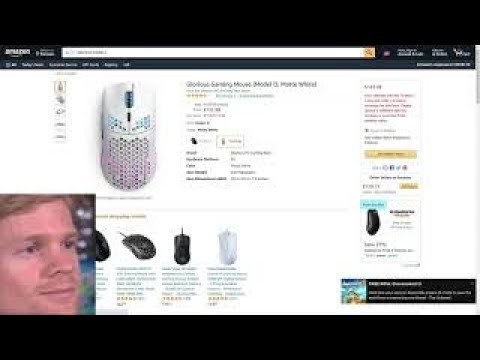The image is a compact, rectangular snapshot of a cluttered computer screen that appears to be zoomed out, making the text and finer details hard to read. At the very top of the screen is a long, empty black bar. Directly beneath it, there’s a white search bar with some illegible text typed into it on the left side, accompanied by a tan search icon featuring a magnifying glass on the right. On the far left of the search bar is an indistinguishable white logo, followed by some tiny, unreadable text, and on the far right, three clickable text elements that are also too small to decipher.

The main portion of the image is dominated by a large, white area filled with pictures of various computer mice. Notably, in the upper left corner, there is a prominently displayed mouse with a white body accented by green and purple dots, though the accompanying description is too blurry to read. Below this mouse is a photograph of a Caucasian man with short brown hair. Adjacent to his image, towards the right, are pictures of several more mice: three are black, one is white, and another black mouse is partially cut off.

Underneath these images is a series of black text lines, which are unfortunately too small to be legible. On the far right, there is a tall white box brimming with text, featuring a noticeable yellow bar with black clickable text. Close to the bottom left of this section is a black mouse and an aqua blue bar with unreadable blue text, accompanied by more small black text next to and below the mouse.

Further down, near the lower right of the image, there is a long, thin black box containing numerous white text elements, all of which are too small and blurry to read. Immediately to the left of this box is a small square with an indeterminate image. Lastly, at the very bottom of the image, there is a long, thin black box that, like the one at the top, is empty.